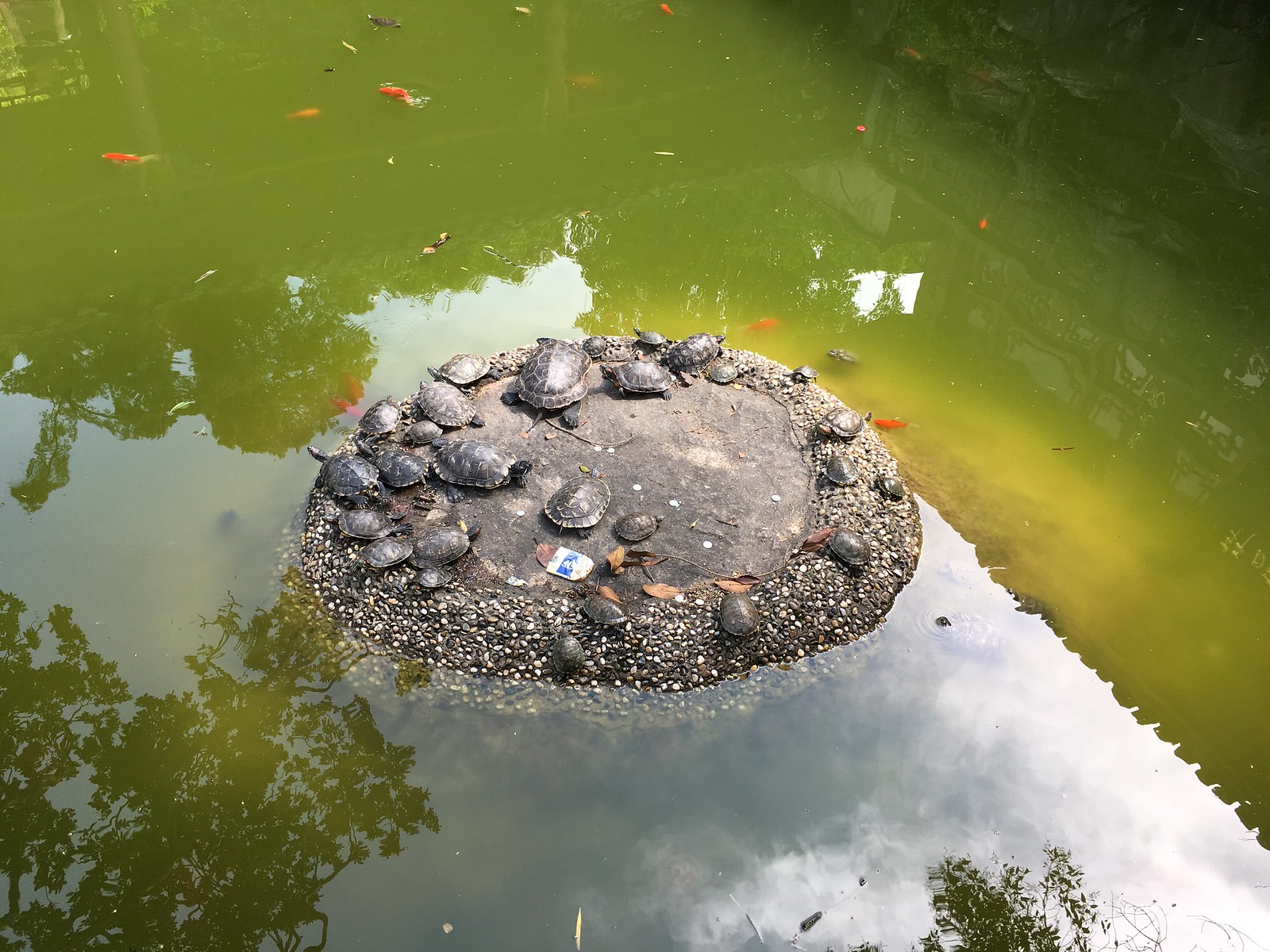A photograph captures a tranquil, murky pond with green and yellowish tinted water that appears stagnant and algae-filled. The water hosts a number of bright orange fish, possibly koi or large goldfish, mingling with a few smaller white and black ones. Prominently featured in the center is a small, man-made concrete island adorned with smaller stones around the rim, providing a perch for numerous dark gray and green turtles of varying sizes. Reflecting the sky above, which is blue with patches of gray clouds, the water also mirrors the surrounding lush green trees. A dark stone retaining wall can be spotted in the upper right-hand corner of the image, enhancing the serene yet slightly overgrown ambiance of this natural setting.